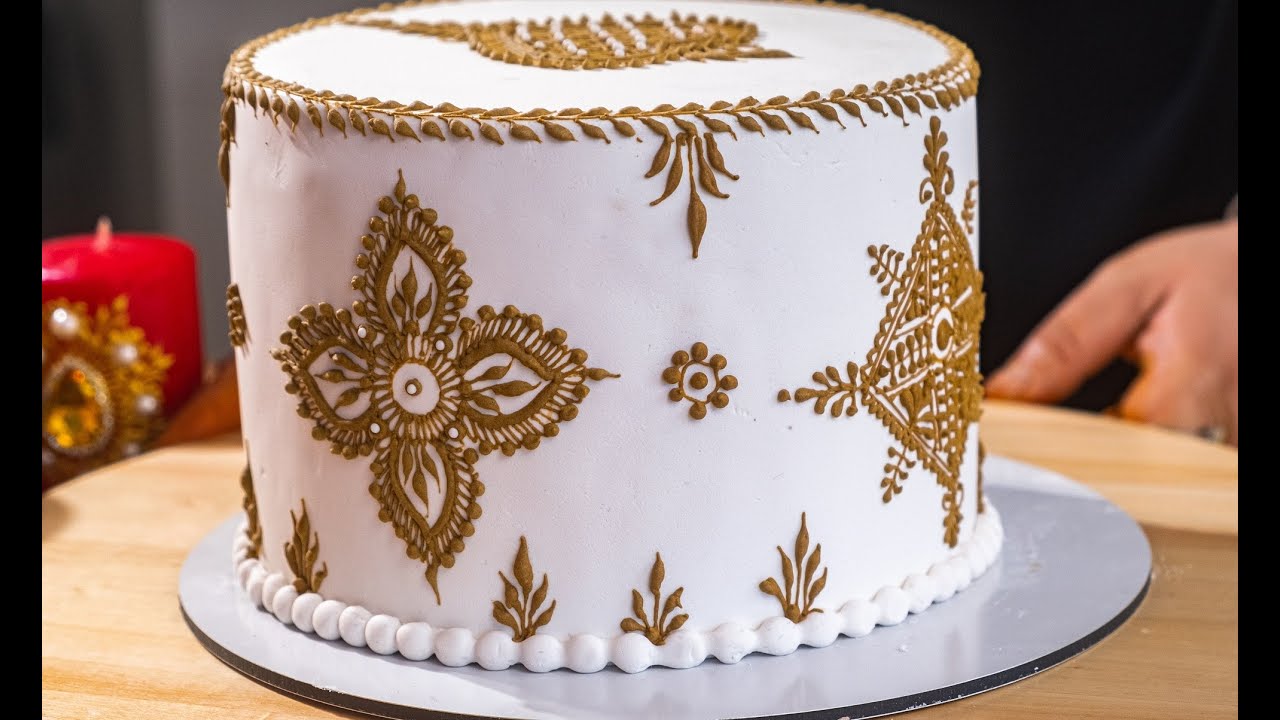The image features a close-up of a circular, white-iced cake adorned with intricate, light brown and golden floral patterns both around its sides and on top. The top of the cake showcases a wreath of golden plants and white edible pearls, crowned by a prominent teardrop-shaped decoration. The base of the cake is encircled by a series of white icing circles, and it sits atop a white platter that is placed on a wooden circular board. In the background, a red candle stands on the left alongside what appears to be a piece of gold jewelry, while a pale or white hand is visible on the right side of the image, seemingly showcasing the cake.